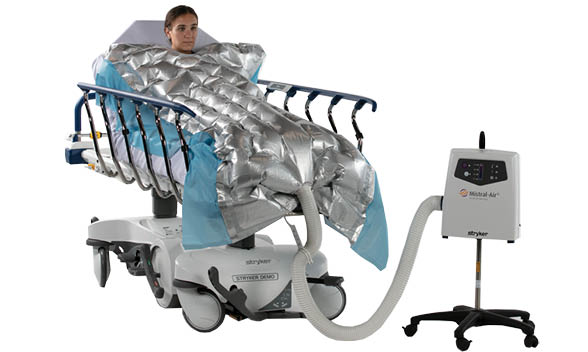In this photoshopped image, a young woman is lying on a hospital bed or medical gurney with raised arms on the sides. She appears to be strapped in and covered by a puffy, shiny silver blanket, which has blue sleeves draping down either side of the bed. The background is entirely white, creating a stark contrast. A gray hose protrudes from the foot of the blanket and connects to a wheeled device, which appears to be labeled "Mistral Air." This machine, with visible buttons, seemingly functions to either provide or compress air, possibly to maintain the blanket's inflated state. At the base of the device, the word "Striker" is also visible.